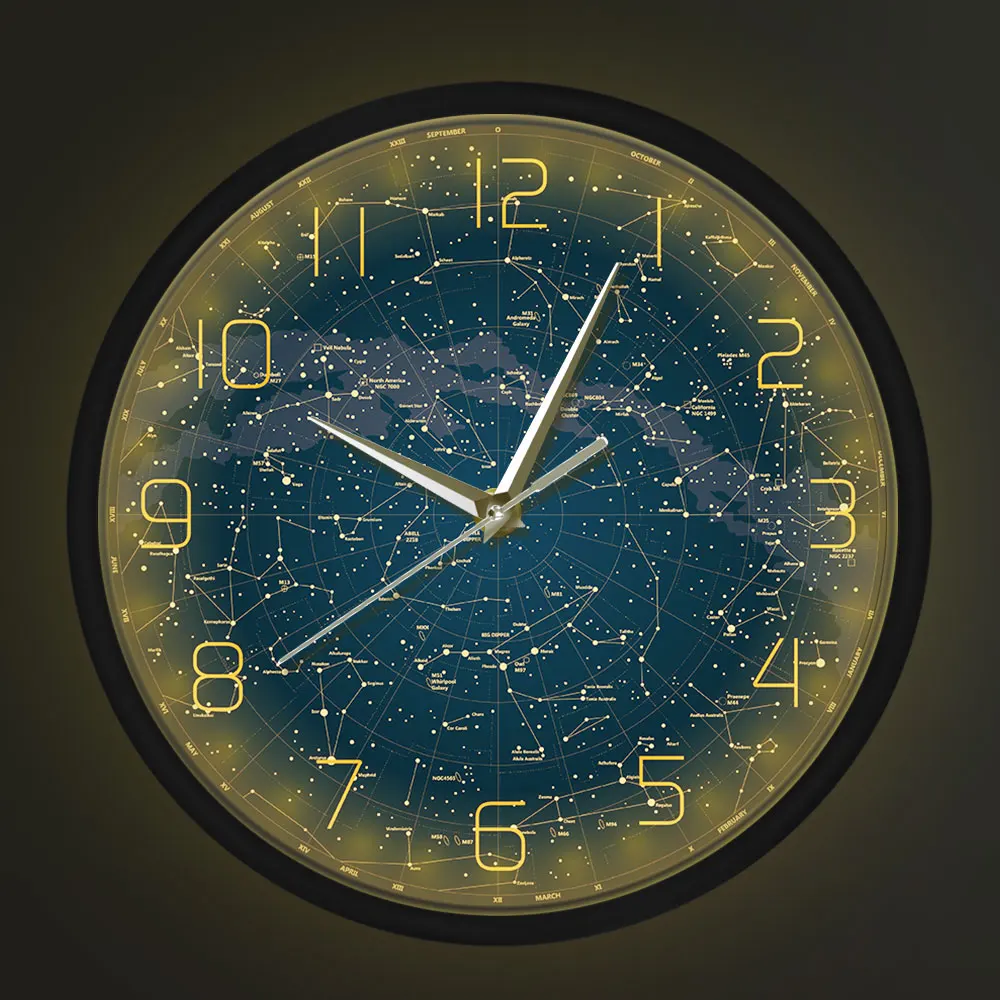This image depicts a sophisticated star clock, which uniquely combines traditional timekeeping with a constellation map. The clock face is bordered in a sleek black and features yellow numbers from 1 to 12, each with yellow lighting around them. The hour, minute, and second hands are metallic silver with dark yellow accents. The interior of the clock displays an intricate constellation map that shows hundreds of stars, indicated by white dots, some of which are connected to form constellations. These constellations are marked clearly, but the text is very small and difficult to read. The background of the constellation map has a dark bluish-gray color and includes subtle cloud-like formations. The clock also has markings for the months around its outer edge, with September at the top, and the other months following in sequence around the clock face. The current time displayed on the clock is 10:04, with the second hand pointing towards 8, the hour hand at 10, and the minute hand just before 1. The overall background of the image features hints of yellow light, but primarily remains a dark gray color.